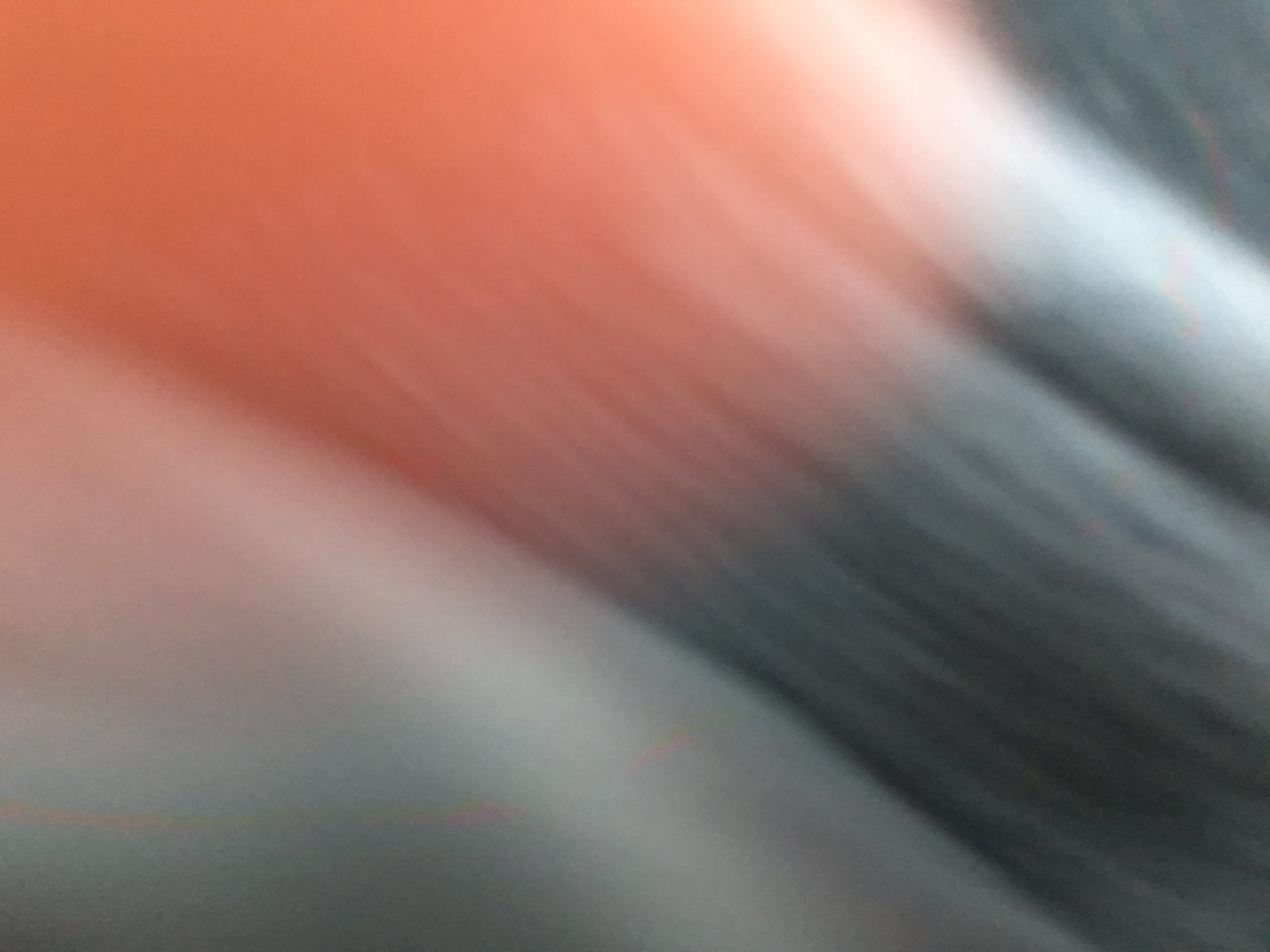A highly abstract, blurry image dominated by a blend of colors. It features a strong presence of reds starting from the left, transitioning into a distinct streak of white. At the top left corner, shades of pink and peach are subtly visible. Below that, towards the bottom left, shades of gray interspersed with white streaks are present. The bottom left corner features a mix of peach, gray, and more prominent white areas. The overall effect is a chaotic but intriguing mix of colors with no discernible shapes or focal points.